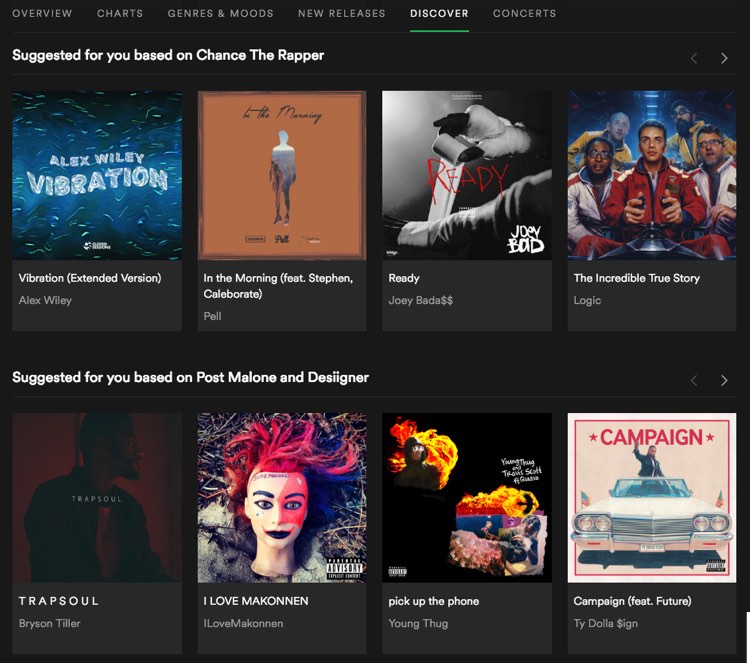Screenshot of a music discovery platform interface with a sleek black background. At the top, a navigation menu displays tabs labeled "Overview," "Charts," "Genres," "Moods," "New Releases," "Discover," and "Concerts," with "Discover" highlighted in green. 

Under "Suggested for You based on Chance the Rapper," four album covers are showcased:
1. "Vibration" by Alex Wiley - Featuring a serene waterscape at the top.
2. "In the Morning" featuring Stephen Colobright by Pell - Boasting a brown background with an image of a person.
3. "Ready" by Joey Badass - Displaying a person's hands against a gray background.
4. "The Incredible True Story" by Logic - Highlighting a group of men intently observing an unseen item in front of them.

Further down, the section "Suggested for You based on Post Malone and Designer" includes:
1. "Trap Soul" by Bryson Tiller
2. "I Love Makonnen" by I Love Makonnen - Featuring a mannequin head with red hair.
3. "Pick Up the Phone" by Young Thug - Set against a dark black background with an image of a person standing in front of a fire.
4. "Campaign" featuring Future by Ty Dolla Sign - Showcasing a white car with a person inside.